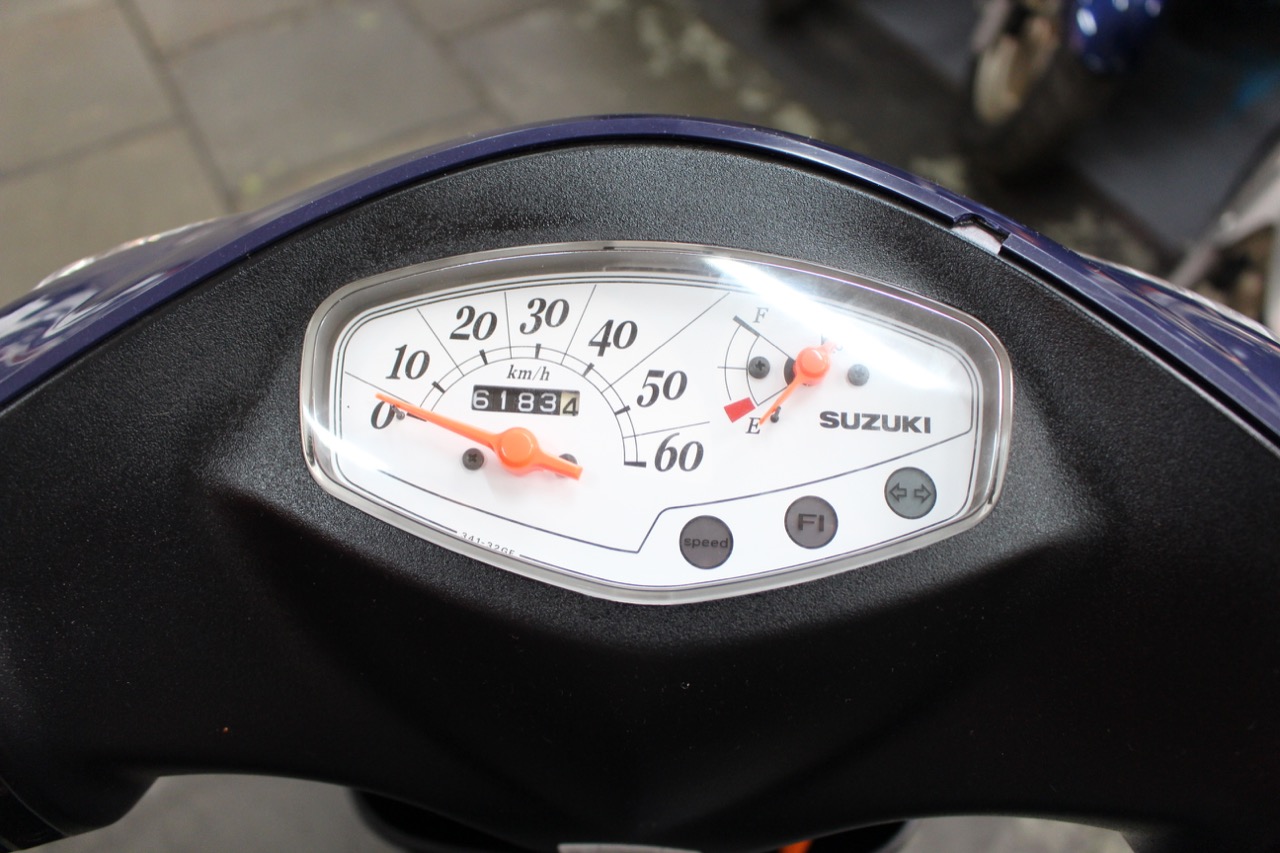This horizontally oriented color photograph showcases the upper section of a Suzuki vehicle, likely a moped or possibly a watercraft. The focus is on the black dashboard, which is encased in a plastic cover over its central part. Prominently featured is a speedometer that maxes out at 60 km/h, with an orange-colored gauge. The odometer reads 6183 kilometers. To the right of the speedometer is a fuel gauge, which is currently pointing below empty, indicating that the machine is off. The empty section of the gauge is marked with a red zone. Beneath these analog meters are three small circular digital displays labeled "Speed," "Fi," and accompanied by arrow icons. The exterior of the vehicle is a blue metallic color, forming an arc that spans from the left middle to the right middle of the image. The vehicle is situated on a brick walkway, and in the blurred background at the top right corner, some chairs or other indistinct objects are visible.